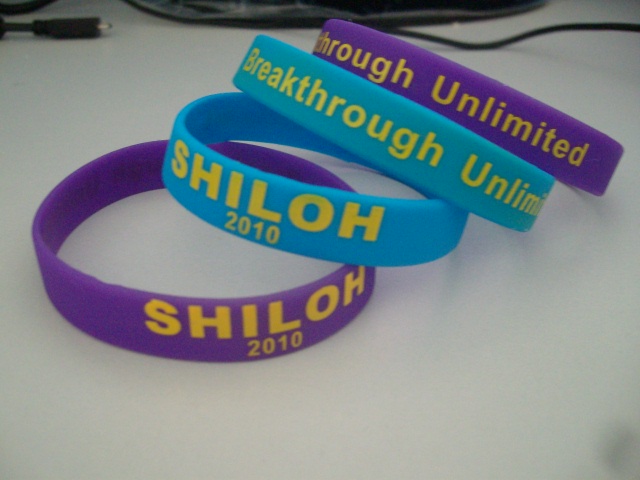The photograph features four rubber wristbands stacked and overlapping on a white flat surface. Two wristbands are purple with yellow text that reads "Shiloh 2010," and the other two are blue (or turquoise) with the same yellow text. One blue and one purple wristband have the words "Breakthrough Unlimited" printed on them. The text on the "Breakthrough Unlimited" wristbands is partially obscured due to the stacking.